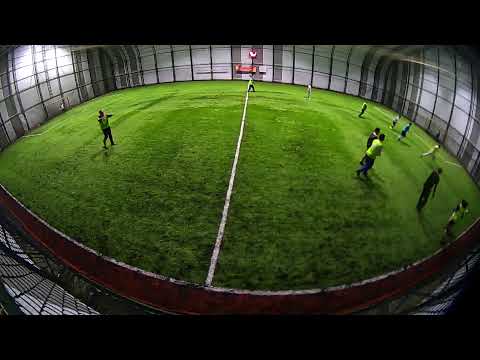The image captures an indoor football pitch with a green playing field, characterized by a circular shape and a white line running through its diameter, emphasizing the field's symmetry. The field is enclosed by light grey walls and a chain-link fence, and the photo's top and bottom edges are marked by a prominent black band, possibly due to lens distortion. There are approximately 10 to 12 people on the pitch, dressed in either black or high-visibility neon green attire, suggesting a casual practice rather than a formal match. A single goalpost is visible in the background, with most players positioned on the right side of the field, some near the goal. The scene appears relaxed and informal, likely representing a recreational activity or a drill session.